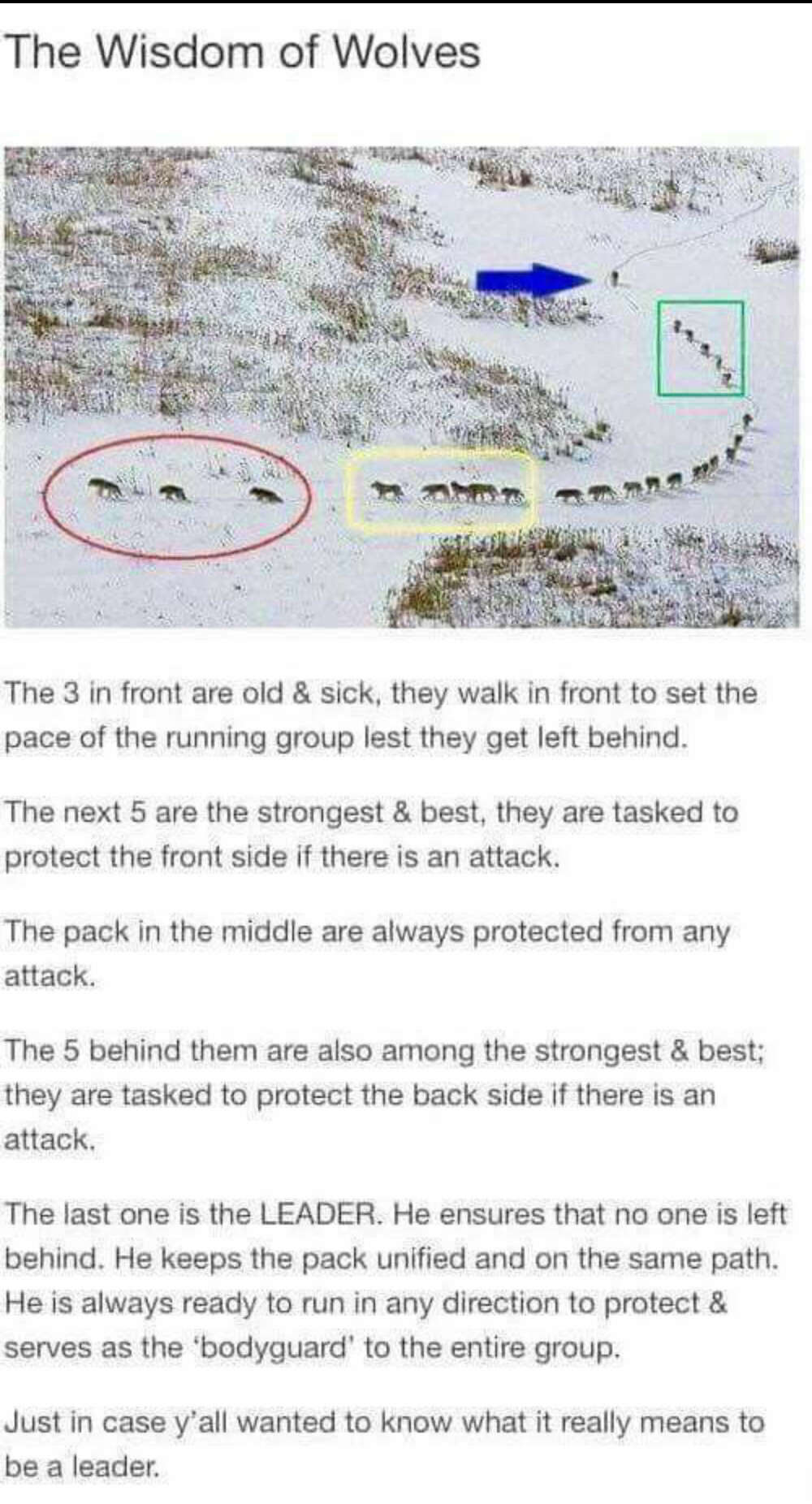The image, titled "The Wisdom of Wolves," depicts a line of wolves traversing a snowy hillside. It features three distinct groups highlighted with colored shapes: the first group of three wolves circled in red, the next five in a yellow box, and another set of five in a green box. An additional blue arrow points to a solitary wolf at the back of the pack. The accompanying text explains the roles of each group: the three wolves in front are old and sick, setting the pace to avoid being left behind; the next five are the strongest, tasked with protecting the front in case of an attack; the central pack is shielded from any attacks; the five behind them are also strong, safeguarding the rear; and the lone wolf at the back is the leader, ensuring no one is left behind and maintaining the group's unity, ready to defend and guide the pack. This setup illustrates a profound lesson on leadership and protection within the wolf community.